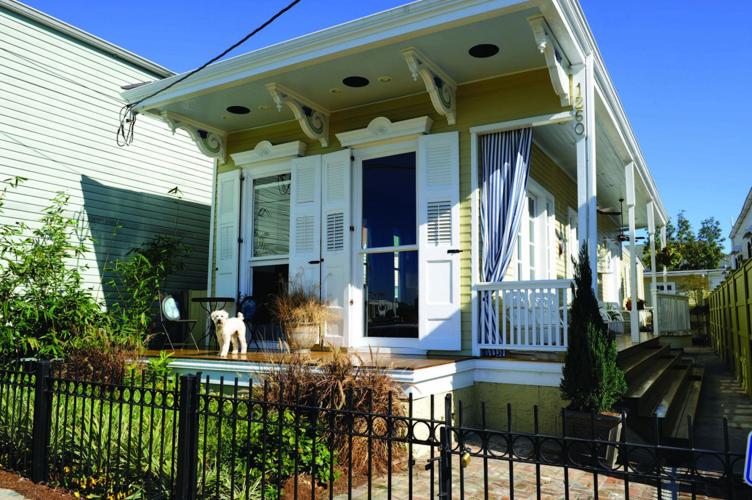This detailed daytime color photograph showcases the front of a mustard yellow shotgun house with white trim, number 1260 on the post, and a wooden porch featuring a small table with two chairs. Standing on the porch, a white dog is looking directly at the viewer. The house has a distinctive black wrought iron fence in the foreground and four long steps leading up to the entrance. To the left, there is a grassy garden area with green and brown plants, and to the right, a small brick patio. The house features large windows with white shutters and storm doors. Behind the house, trees and a clear blue sky provide a picturesque backdrop. A walkway leads toward the back, and to the left of the house stands another building with a white roof, appearing square in shape from the perspective of the image.